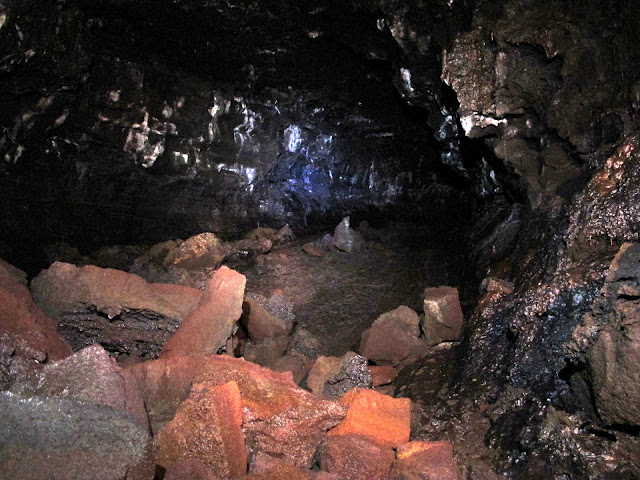The photograph captures the interior of a dark, mysterious cave, likely near its entrance. The image features predominantly dark gray and black rocky walls, which become increasingly shadowed as you move further into the cave. In the foreground, a mix of vibrant reddish-orange rocks is prominently illuminated, possibly by the camera's flash. The rocks appear jagged and broken, with some having a sparkly, crystal-like quality that reflects light, giving them a shiny appearance. The floor of the cave is littered with these rocks, forming piles that contrast against the darker surroundings. There is an impression of moisture on some of the surfaces, which adds to the glistening effect. Additionally, subtle hues of purple and bluish tones are visible on the rocks, suggesting reflections or minerals within the cave walls. The overall ambiance is one of intrigue and rugged beauty, hinting at a place possibly used for mining or exploration.